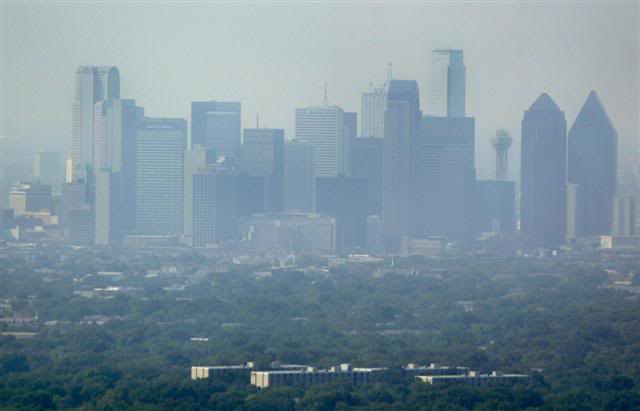This aerial photograph captures a dense cityscape shrouded in hazy, smog-laden air, rendering the scene somewhat blurred and gloomy. Dominating the skyline are an array of skyscrapers in varying shapes and sizes. Some buildings are simple rectangles, while others are more complex, with triangular tops and differing widths and heights. The cityscape towers over a foreground rich with greenery; vast wooded areas and forests interspersed with smaller buildings. These structures are mostly rectangular, apartment-like buildings that stand in stark contrast to the towering skyscrapers in the background. The overall cityscape blends into a murky, grey sky, hinting at pollution or heavy fog, and creating a subdued, almost monochromatic palette for the photograph.